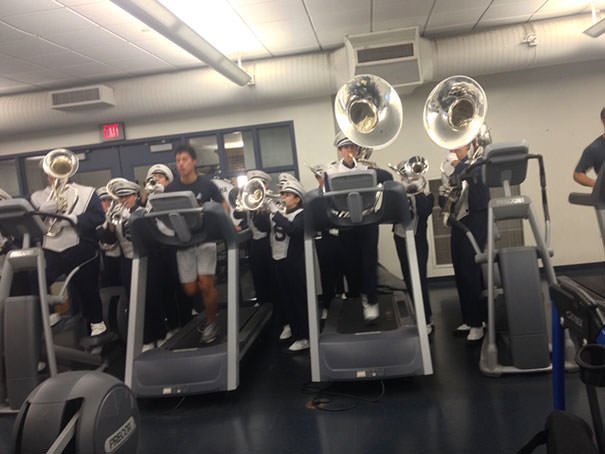The image is a slightly tilted rectangular shot capturing a unique scene in a gym setting where members of a marching band are practicing on treadmills. The angle of the photo is approximately 40 degrees from left to right. In the foreground, four treadmills are aligned facing forward. The first treadmill on the left is occupied by a band member whose face is obscured by a brass instrument. This person, dressed in a white-and-black marching band uniform with distinctive white socks over black shoes, appears to be a trombonist or similar brass instrument player. 

Next to this band member is an individual not in uniform, engaged in a workout. Adjacent to this person is a man playing what appears to be a tuba, a large brass instrument, while standing behind the treadmill. Beside the tuba player is another tuba player also standing, with his instrument slightly angled towards the left. 

In the background, more band members holding brass instruments, potentially tubas and trombones, are seated or standing, creating a bustling scene of preparation and exercise. The gym is equipped with various exercise machines, and a treadmill and an ambiguous exercise machine are spotted in the lower left corner. 

On the far right, half of a person in a mid-range blue shirt and white pants appears to be standing near another machine, possibly another treadmill. The room features fluorescent lighting, a black shiny floor, ceiling tiles, a large white wall in the back with an exit sign, and a doorway with glass windows and doors leading to a hallway.

This detailed scene captures the juxtaposition of a traditional marching band setting within the modern environment of a gym, highlighting the unique methods of their practice and preparation.